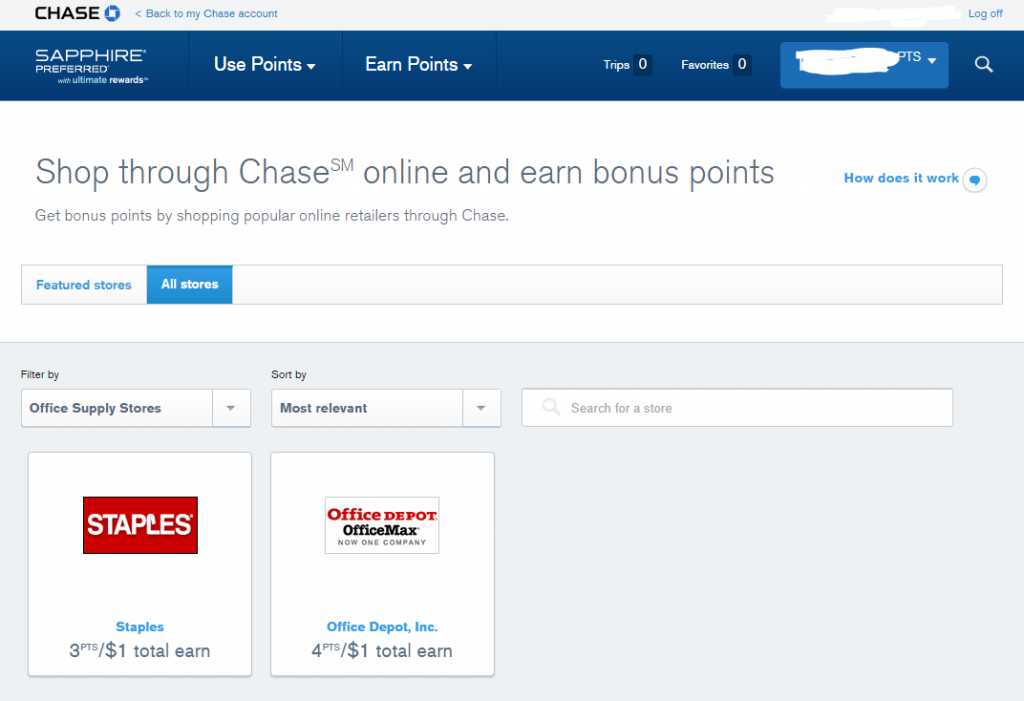**Screenshot Description:**

The image is a screenshot featuring a gray background and appears to be from the Chase online account interface. At the top, there are navigation options labeled "Chase back to my Chase account" and "Log off." The interface displays several tabs including "Sapphire Preferred," "Use Points," "Earn Points," "Trips," and "Favorites." There is also a word that is censored or whited out.

Underneath these tabs, a search bar is visible along with a prompt to "Shop through Chase online and earn bonus points." A brief explanation states that users can earn bonus points by shopping at popular online retailers through Chase. A hyperlink titled "How does it work?" in blue suggests additional information can be accessed.

The interface includes a chat icon and two sections: "Featured Stores" and "All Stores." Additionally, there are multiple filter options including "Filter by" which focuses on "Office Supply Stores" and "Sort by most relevant." Another search bar is available for further search refinement.

Highlighted within the screenshot is a red rectangle containing "Staples" displayed in white text, with "Staples" also written in blue text below. Information about the points system is shown, indicating "3 PTS / $1 total earn." Similarly, "Office Depot" and "Office Max," now one company under "Office Depot Inc." is mentioned, offering "1 PT / $1 total earn."

Overall, the image portrays an interface design for managing points and rewards while shopping through Chase's online platform.